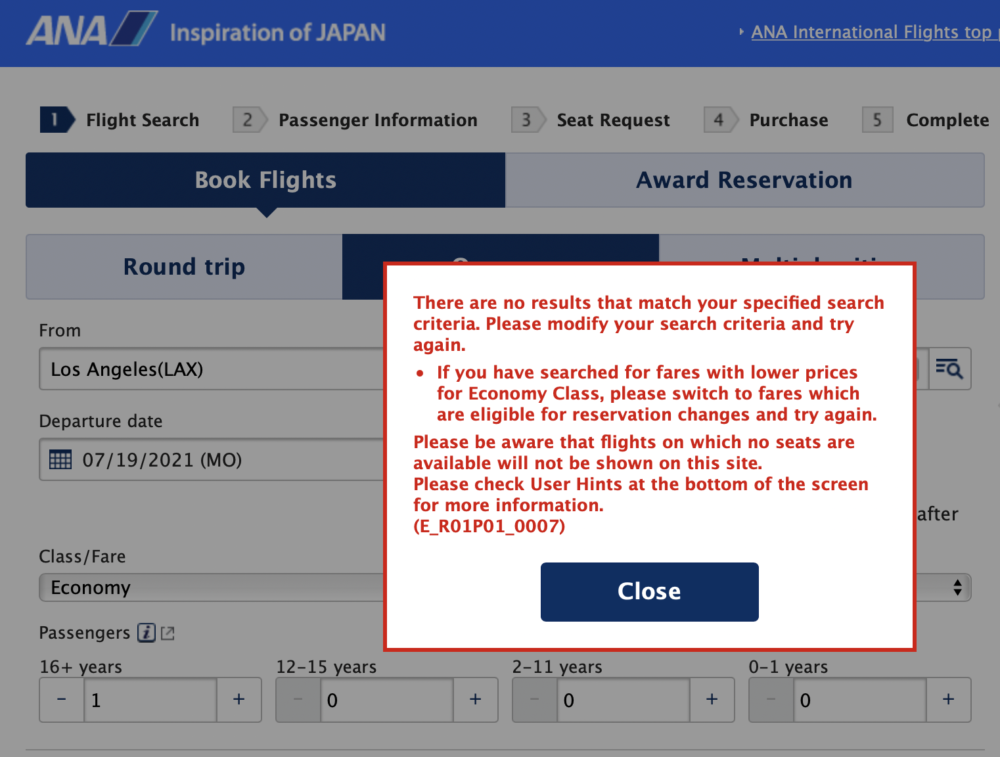The image showcases a travel booking website, with the primary background grayed out to bring attention to a pop-up window in the foreground. The pop-up is dominated by text in red, indicating an error message from ANA (All Nippon Airways), which is branded as "Inspiration of Japan." The central message in the pop-up reads: "No results match your specified search criteria. Please modify your search criteria and try again."

Highlighted within the pop-up are additional details, including a black or red circle icon, and a smaller text specifying that the user has searched for cheaper fares in the economy class. The message advises switching to fares that are eligible for reservation changes. Another warning explains that flights with no available seats will not be displayed on the site and recommends checking user hints at the bottom of the screen for more information. At the bottom, a reference code reads "(e_r01_p01_0007)." A prominent blue button labeled "Close" is visible at the bottom of the pop-up.

Behind the pop-up, partially obscured, is the main site navigation showcasing the steps involved in booking a flight. These steps include:
1. Flight Search
2. Passenger Information
3. Seat Request
4. Purchase
5. Complete

The interface shows that the user is on the "Book Flights" tab, marked in dark blue, with an adjacent tab labeled "Award Reservation." Below the main navigation tabs, the user has selected a "Round Trip" option. Also partially visible are details from the search criteria, including "from Los Angeles," a departure date, and the selected economy class for a single passenger aged 16 or older.